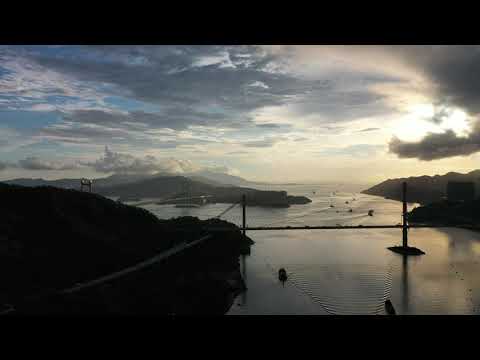The image captures a dark, moody scene near a body of water, possibly a bay in California. The water appears shallow, close to the shore, with various objects protruding from it, and boats navigating through. The center features a suspension bridge, likely the Golden Gate Bridge, with its two prominent beams towering on either side. The atmosphere suggests a pending storm or dusk, with the sky dominated by dense clouds, allowing only slivers of blue to peek through. The left-hand side reveals a tree-covered hill, and distant, shadowy mountains frame the background. The overall tone is somber, accentuated by the overcast, brooding sky and a dark rectangular border outlining the image.